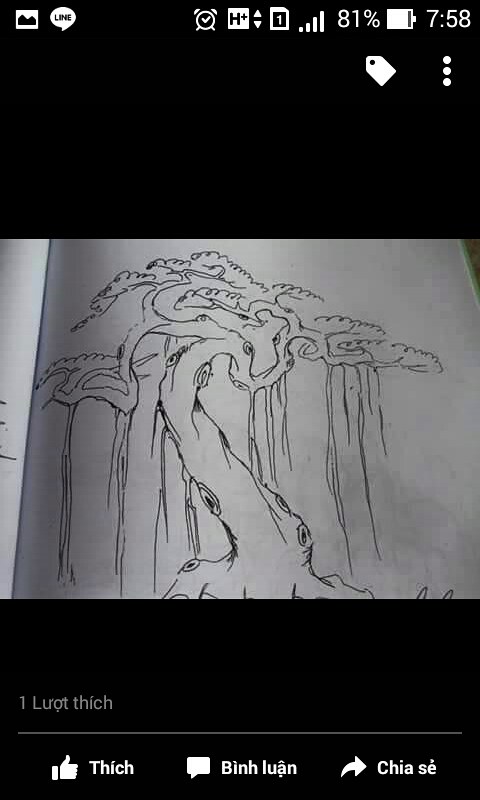Image Description:

A detailed sketch of a tree dominates the center of the image, with intricate, curvy lines that represent the tree trunk and branches spreading out towards the top. The branches have multiple lines dripping down, resembling vines or elongated leaves, and the sketch is rendered on light gray paper.

The image appears to be a screenshot from a social media post in a foreign language. At the very top of the screen, a series of cell phone icons are displayed in white against a black background: 

- Starting from the left, there is a gallery icon.
- Next to it is a messaging icon labeled "Line."
- Following is an icon resembling an alarm clock.
- Next in line is a signal indicator labeled "H+."
- An upward arrow and a downward arrow icon are placed beside the signal indicator.
- Adjacent to this is a white square with the number "1" inside.
- Moving right, there is a Wi-Fi signal icon.
- Further to the right, the battery percentage, "81%," is shown.
- Near the battery percentage is almost a fully shaded bar indicating battery level.
- Finally, the current time displayed is "7:58."

Below these icons and in a black background, there are an editing icon and a three-dot menu option. At the bottom of the image, also against a black background, three options are available in a non-English language.

Overall, the image combines elements of a hand-drawn tree sketch with a digital user interface, contextualized within a social media application.